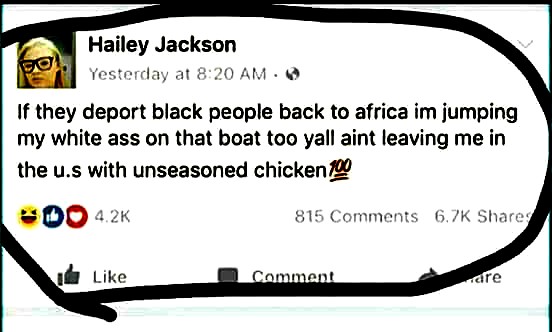In this widely-shared social media post by Hayley Jackson, depicted in a mobile screenshot, Hayley is seen with long blonde hair and black glasses in her thumbnail avatar. The post, which has been manually circled with black marker, was published yesterday at 8:20 AM. It humorously reads, "If they deport black people back to Africa, I'm jumping my white ass on that boat too. Y'all ain't leaving me in the U.S. with unseasoned chicken. 💯" The post went viral, garnering 4.2K reactions—ranging from likes to heart emojis—815 comments, and an impressive 6.7K shares, highlighting its significant popularity and engagement online.